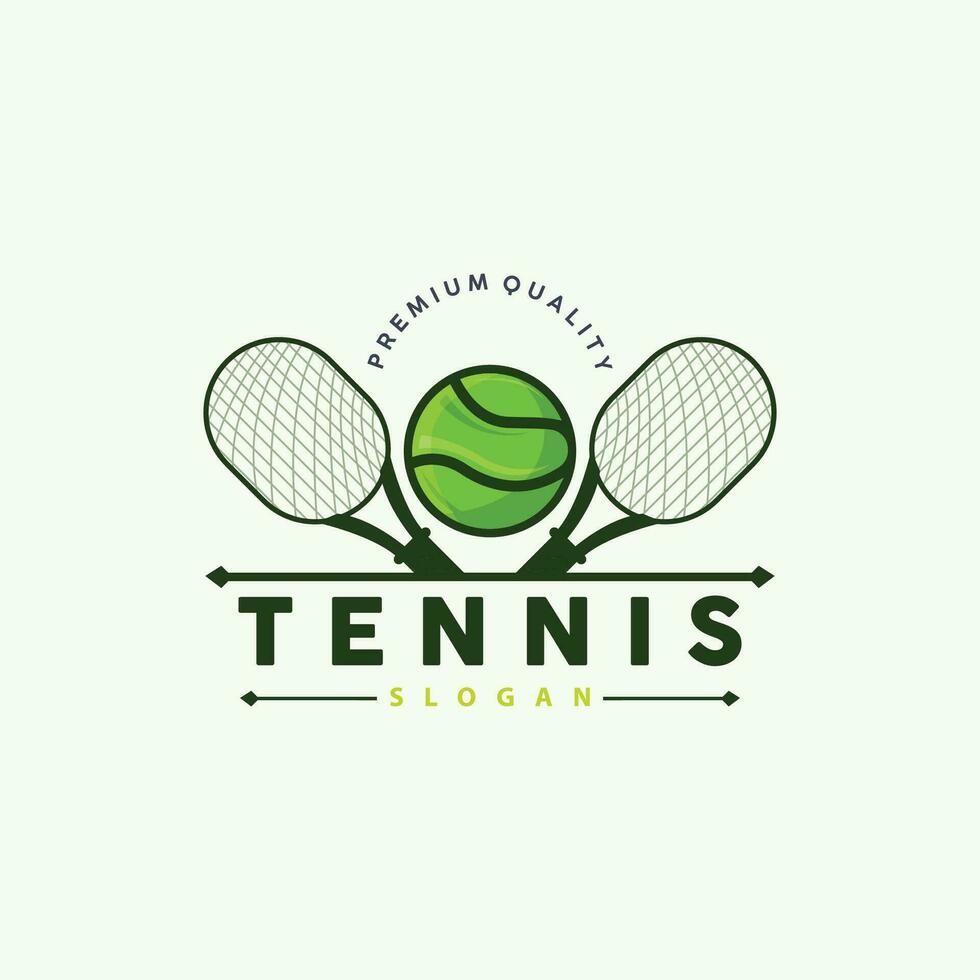The image displays a meticulously designed logo for a tennis-related company or club, set against a pale mint green background. At the top of the logo, the phrase "Premium Quality" is written in a black arching text. Below this, a darker green tennis ball is centered, flanked by two outward-facing tennis rackets. Beneath the tennis ball and rackets, the word "Tennis" is prominently featured in bold, capitalized black letters. Directly under "Tennis," the word "Slogan" appears in a smaller, lime-colored font, with thin arrows extending horizontally from each side. The overall design appears carefully crafted, leaving room for customization such as replacing "Tennis" with the company name and "Slogan" with the organization's specific tagline.